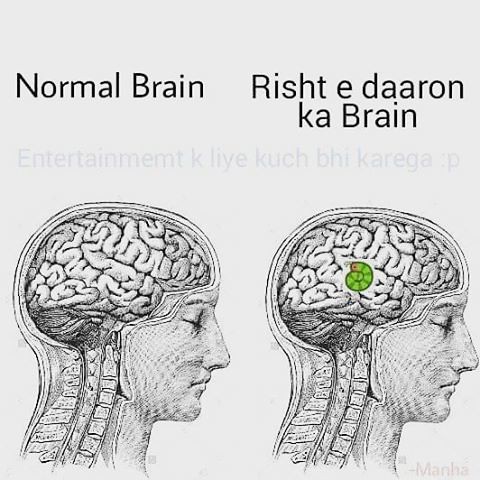The image features a light gray background and depicts a detailed informational chart with two side-view illustrations of human heads showing the brain and spinal column. On the left side, the diagram is labeled "Normal Brain" in clear black font, showcasing a regular brain. On the right side, a similar illustration contains a small, stylized green cartoon worm in the middle of the brain, and is labeled "RISHT-E DARAAN KA BRAIN" in a foreign script that appears to be less easily recognizable. Above this image, in a lighter, more difficult-to-read gray font, there's another line of text reading: "ENTERTAINMENT K LE LIYE KUCH BHI KAREGA" followed by a colon and the letter "P", which might suggest an emoji face. At the bottom of the image, a light brown signature appears, reading "MANHA." The origin of the informational card is not discernible from the image alone.